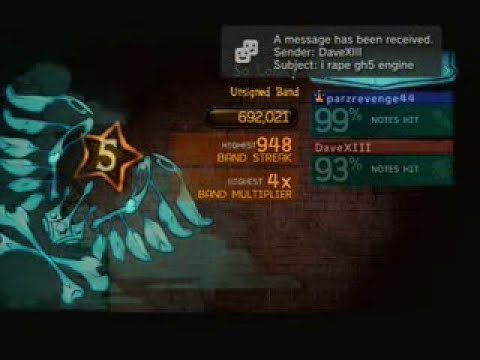This image appears to be a screenshot from a video game, specifically a rhythm game such as Rock Band or Guitar Hero. The background is black with several informational overlays. At the top, there is a gray text box with two theater masks and text indicating that a message has been received from sender "Dave XIII" with the subject "I rape GH5 engine." 

The central part of the image showcases the game results displayed over what seems to be a brick wall background. Dominating this section is a stylized emblem featuring a golden star with the number 5 in the center, flanked by what resembles bones and feathers, and a skull with crossbones beneath it, possibly adorned with wings.

Below the emblem, there's a black box with yellow text showing the number 692,021, likely the score. Further down, a gray text box reveals stats such as a "948 Band Streak" and an "x4 Band Multiplier." To the right, additional statistics are displayed, including "99% notes hit" for one player and "93% notes hit" for another. These details suggest the high achievement levels of the players.